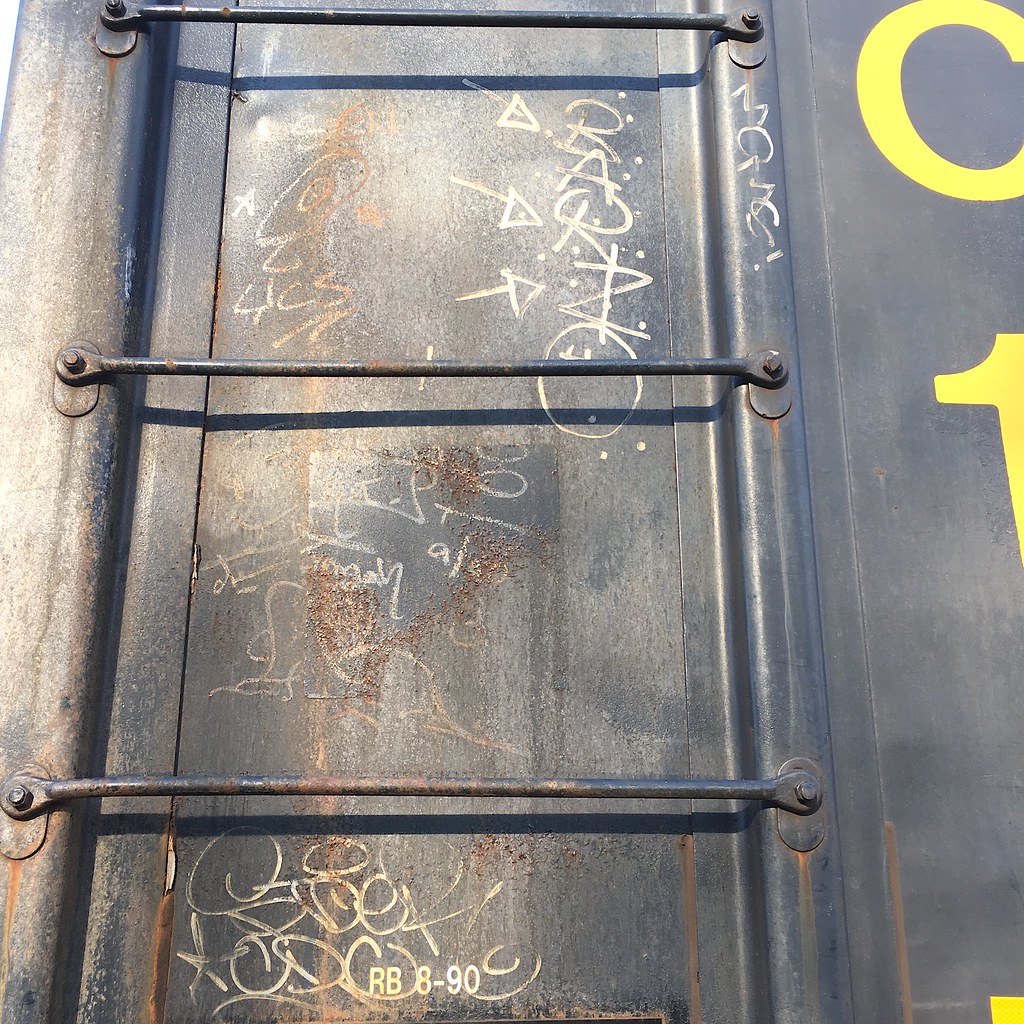This image depicts a close-up view of the side of a train boxcar, primarily focusing on a section with a metal ladder. The dark gray to navy blue steel boxcar is speckled with rust stains and adorned with illegible white graffiti, consisting of arrows, circles, and random letters. Three thin, horizontal rungs of the ladder are visibly bolted onto the structure, indicating it's a climbable feature on the train car. Prominent yellow lettering on the right side spells out a large "C" and a partially visible "1", hinting at some form of identification. Additionally, at the bottom of the scene, the printed label "RB 890" is clearly seen. Illuminated by what appears to be daylight, the weathered and worn appearance of the boxcar tells a story of heavy usage and exposure to the elements.